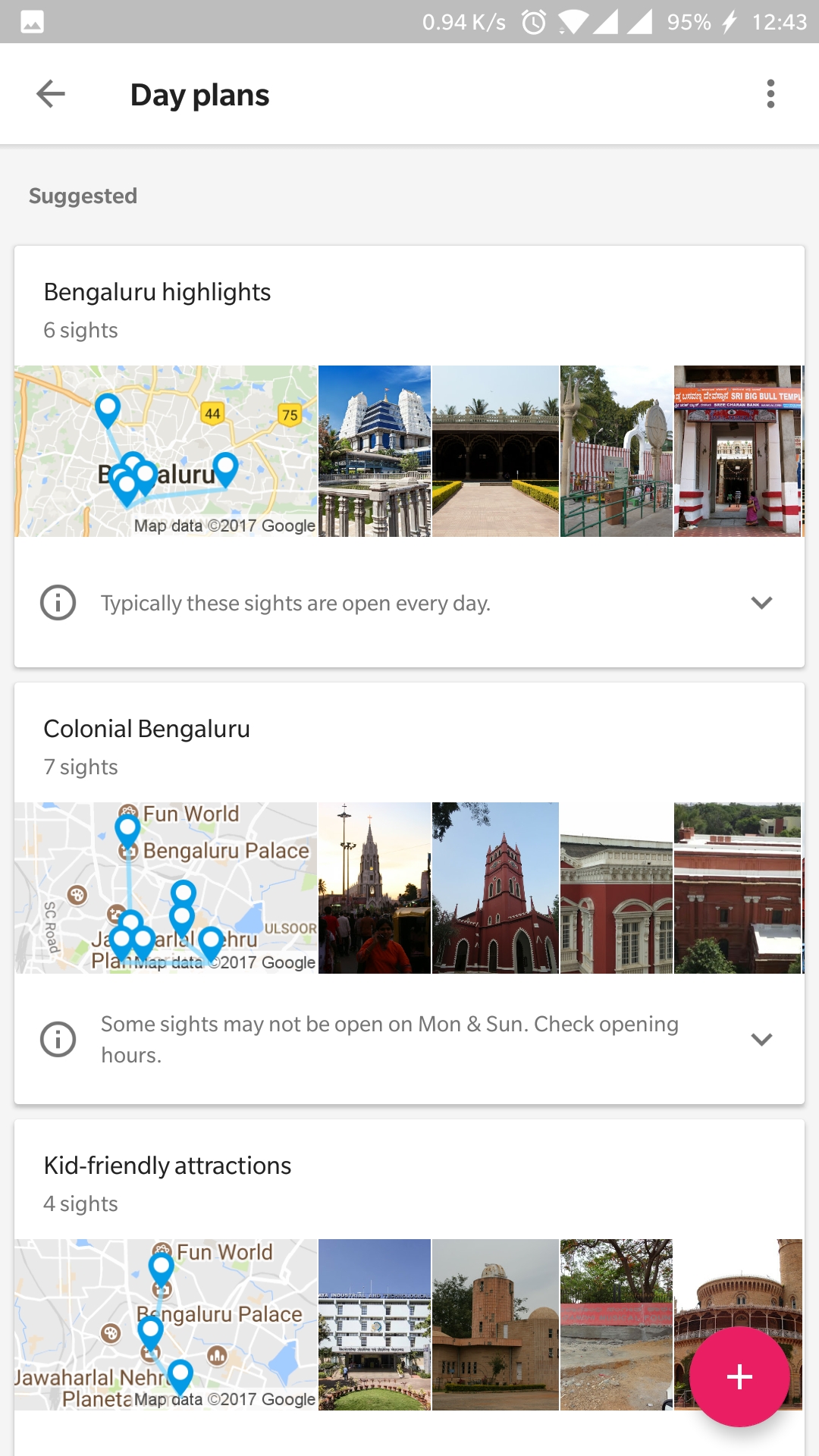This screenshot is captured from an Android mobile device, evident from the status bar at the top. The status bar includes a screenshot icon in the upper left corner, suggesting that the current image is indeed a screenshot. The presence of two reception icons indicates the device supports dual SIM functionality. Additionally, icons for cell signal, Wi-Fi signal, and the current time, shown as 12:43, are visible. The battery icon displays 95% with a lightning bolt, meaning the device is charging.

The main content below the status bar showcases a predominantly white background. At the top, the text "Day Plans" is prominently displayed in black. Beneath this, the section labeled "Suggested" contains three vertically stacked sections.

1. The first section is titled "Bengaluru Highlights," featuring six sites marked on a small map with six blue pins. To the right are four thumbnail images corresponding to these locations.

2. Following that, the section "Colonial Bengaluru" lists seven sites, also marked with seven blue pins on another map. This section includes four thumbnail images to the right of the map.

3. The final section is named "Kid-Friendly Attractions," highlighting four sites, reiterated with four pins on the map and accompanied by four thumbnail images.

Each section provides a visually organized overview of different plans and attractions, with maps and images for easy reference.